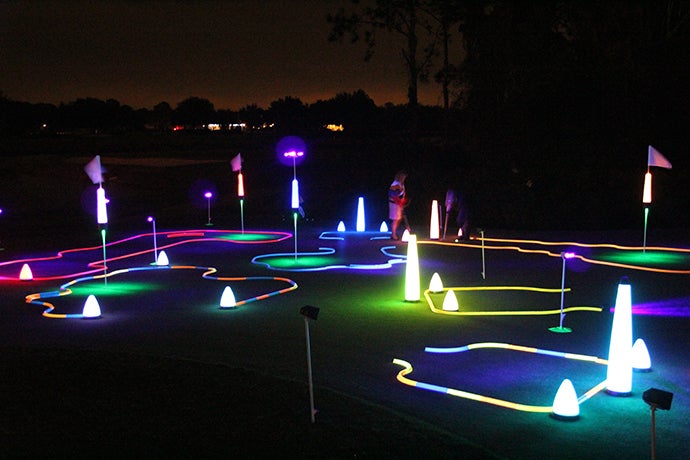The image captures a lively and unique nighttime putt-putt golf course, bathed in a vibrant array of glow-in-the-dark neon lights. Each miniature hole is outlined with fiber optic lights that glow in striking colors such as blue, yellow, hot pink, neon purple, and a green hue illuminating each hole, guiding where the ball should go. Flags are strategically placed at different points across the course, adding to the playful and inviting atmosphere. The course's pathways are highlighted by streaks of white neon lights running in various directions. Two people are visible in the distance; one appears to be a lady wearing a skirt or shorts and an elbow-length shirt, suggesting a warm summer night, while the other seems to be a gentleman bending down, possibly adjusting his putt. Surrounding the course are faint lights from nearby homes and the indistinct silhouettes of trees, enhancing the scene's nocturnal charm. The overall setting suggests a delightful and visually stimulating experience, perfect for enjoying a night of miniature golf.